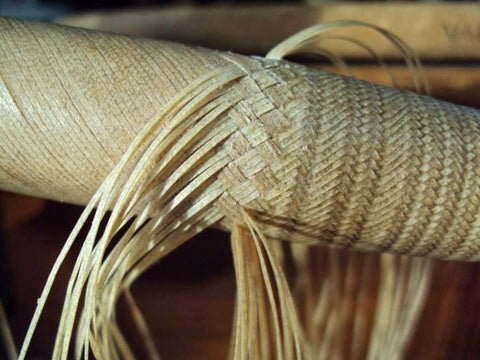This photograph captures a close-up view of an unfinished weaving project, likely using straw or rattan material. The image focuses on a cylindrical shape which is being intricately woven with a zigzag diamond pattern. The right side of the cylinder showcases the more finished sections, exhibiting a tightly interlocked design. In contrast, the left side displays the initial stages of the weaving process, where long strands are yet to be fully integrated. The woven layer adds a decorative touch over a base layer that runs vertically upward at an angle. The background, slightly blurred, hints at an indoor setting, possibly a workshop with wooden tables and various objects.